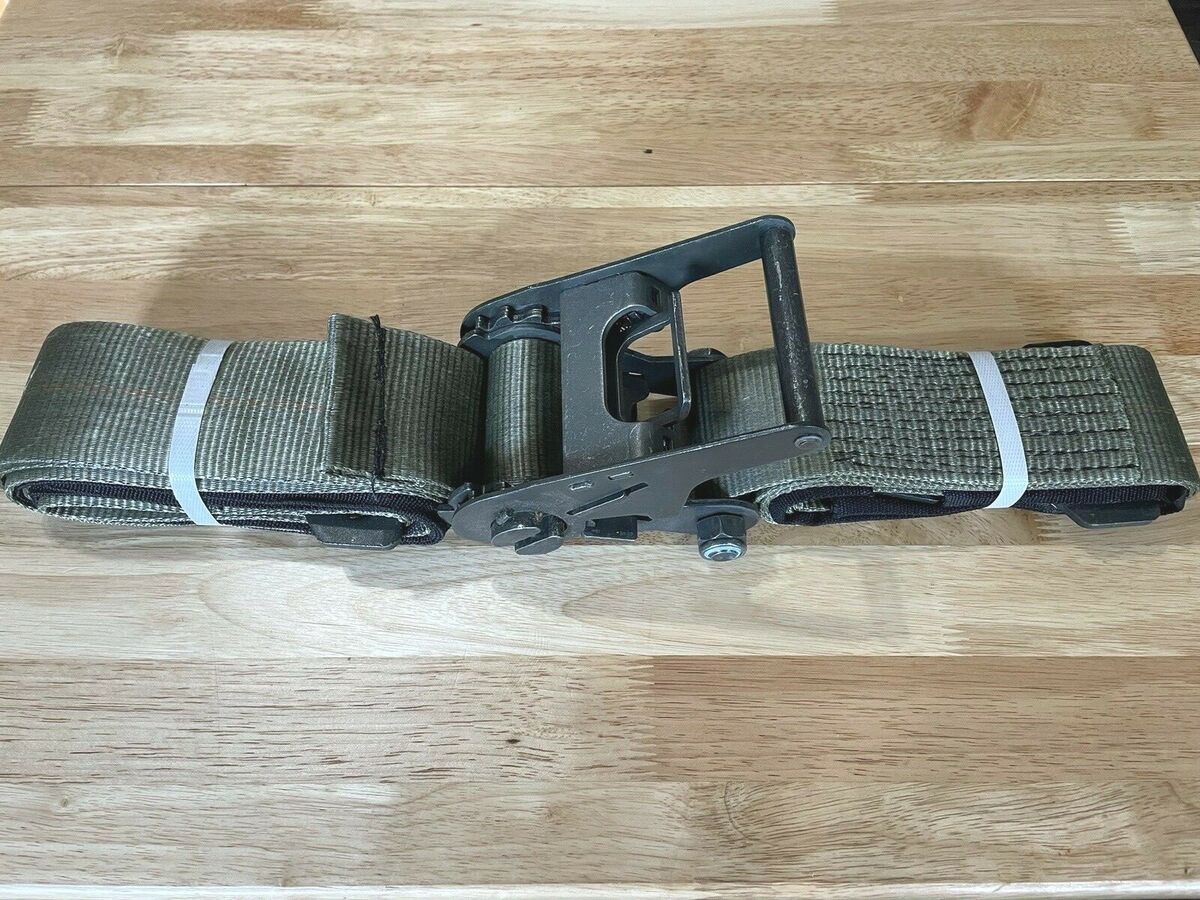The image depicts a black seatbelt-like strap made of thick, woven fabric resting on a light brown wooden surface, possibly a table or floor. The strap is secured at both ends by white plastic bands to prevent it from unravelling. At its center, there is a robust-looking black buckle, which is either metal or hard plastic. The buckle is attached securely, suggesting it is functional and possibly used for securing an object or person. The photograph appears to have been taken in landscape mode with natural light seemingly coming from the left, illuminating parts of the wooden background.